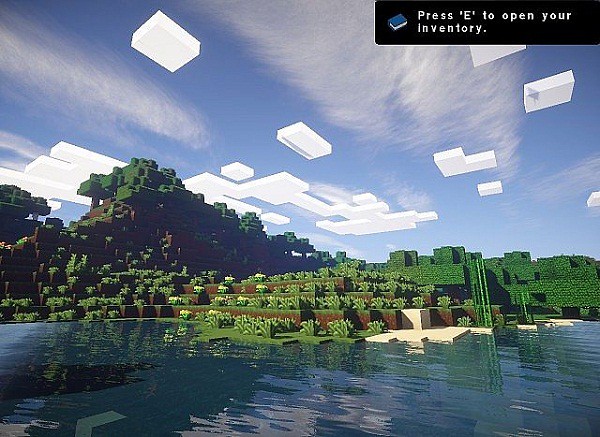This detailed caption portrays a Minecraft game screenshot:

The image displays a Minecraft game screen. In the top right corner, there's a black rectangular box with white text saying "Press E to open your inventory" next to a blue and white book icon. The foreground is dominated by a body of blue water. Centrally, there is terraced landscaping that extends into the water, resembling an amphitheater with layers of greenery supported by brick walls. This central ground features square-shaped plants and bushes typical of Minecraft's blocky aesthetic. On the left side, a mountain is visible, topped with green, pixelated, square-box trees. The sky is a baby blue, adorned with bright white, square-shaped clouds and slightly dimmer floating white boxes beneath them, maintaining the game's signature 8-bit, pixelated style.